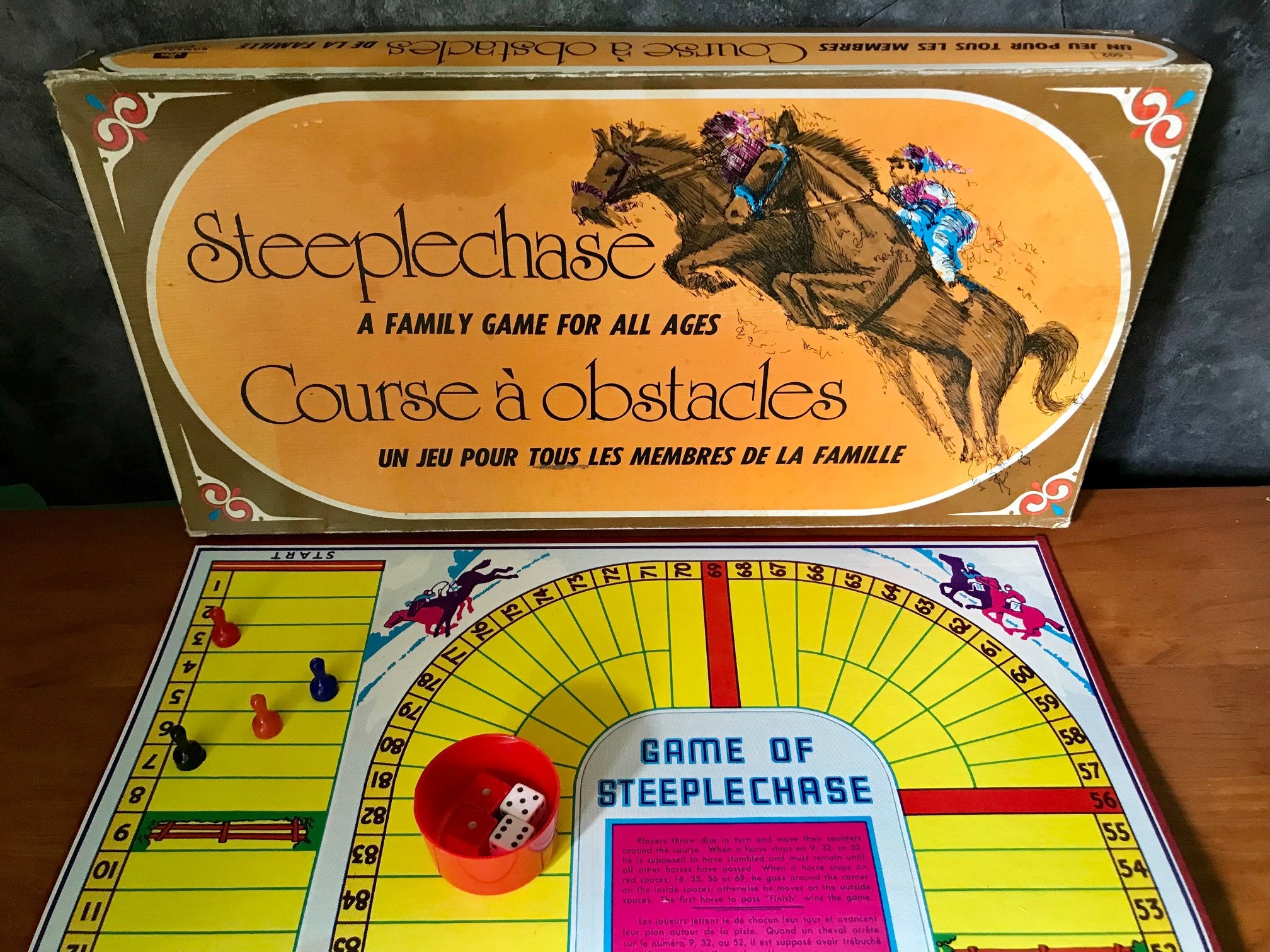This photograph features a vintage board game called Steeplechase: A Family Game for All Ages (with additional French text on the box). The game, which clearly shows signs of age through the wear on the edges of its box, is set up on a wooden desk. The box itself, featuring an illustration of two racing horses with riders in blue attire, stands upright at the back of the photograph. The game board, laid out flat on the desk, is primarily in gold and depicts an oval racetrack numbered from 53 to 84 with an open center. The playing pieces include small plastic horses and a red shaker cup containing dice. Additional elements on the game board include explanatory text and yellow sections. The setup also includes a glimpse of a blue couch and a plain wall behind the desk, enhancing the nostalgic ambiance of the scene.